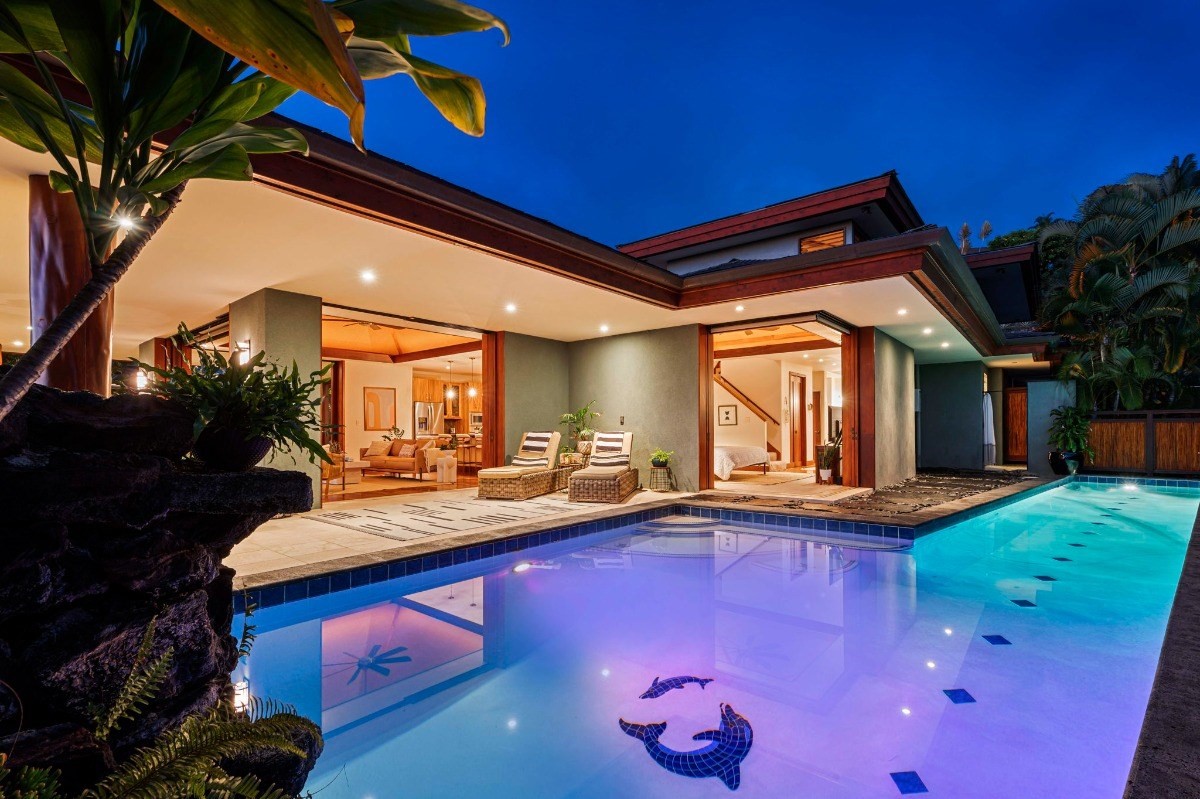This image captures a stunning nighttime view of a luxurious, modern house, showcasing its expansive backyard and beautifully illuminated in-ground swimming pool. The photograph is taken from the opposite end of the pool, which is rectangular with a unique square cutout on the upper left. The pool bottom features intricate tile designs of two dolphins swimming in a circle, accompanied by diamond shapes along the right side, where one might swim laps. The pool's underwater lights cast a mesmerizing array of purples, blues, and greens, enhancing the clear water's allure under a dark, royal blue sky.

The house, primarily one story with a notable two-story section to the right, is finished in white with abundant wood accents. Inside, visible through large windows, the aesthetic includes brown furniture, white walls, wooden floors with throw rugs, and modern lighting fixtures such as can recess lights and pendant lights. The home’s open design extends to the outdoors, seamlessly integrating with the patio area that surrounds the pool.

The patio features sophisticated wicker and wood reclining chairs and various benches set amidst tropical plants and palms. A brown fence and more greenery form the background, while a prominent palm tree on a stone platform stands in the left foreground. Additionally, an overhang with lights extends over the seating area, contributing to the inviting and tranquil atmosphere of this lavish outdoor space.